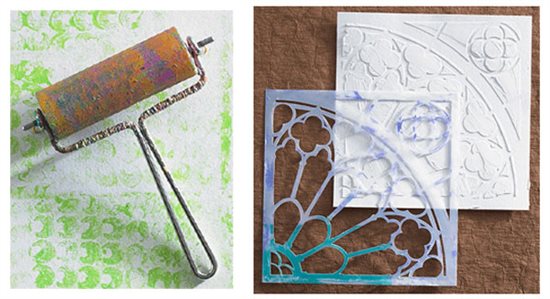The image presents two distinct photographs side by side, both depicting tools and materials used in a craft or decorative painting process. On the left, we see a paint roller stained with a spectrum of subdued colors—purple, orange, blue, and lavender—resting on a white background adorned with a light leafy green, crescent moon pattern. The paint roller's metal frame and handle are positioned with the handle in the lower right corner, extending diagonally left to the middle.

The right photograph showcases a stencil and a ceramic or paper tile placed atop a textured brown surface that might resemble rocky flooring or brown wrapping paper. The stencil, previously white but now marked with paint stains in blues, purples, and whites, features a latticework design incorporating quarter-circle shapes with intricate lace patterns and small heart motifs at the edges. This stencil has been used to transfer its design onto the underlying white tile, which appears pristine apart from the crafted imprints. The tile exhibits various patterns, including club-like symbols and circular forms with semicircular details, highlighting the intricate work achieved through the stencil.